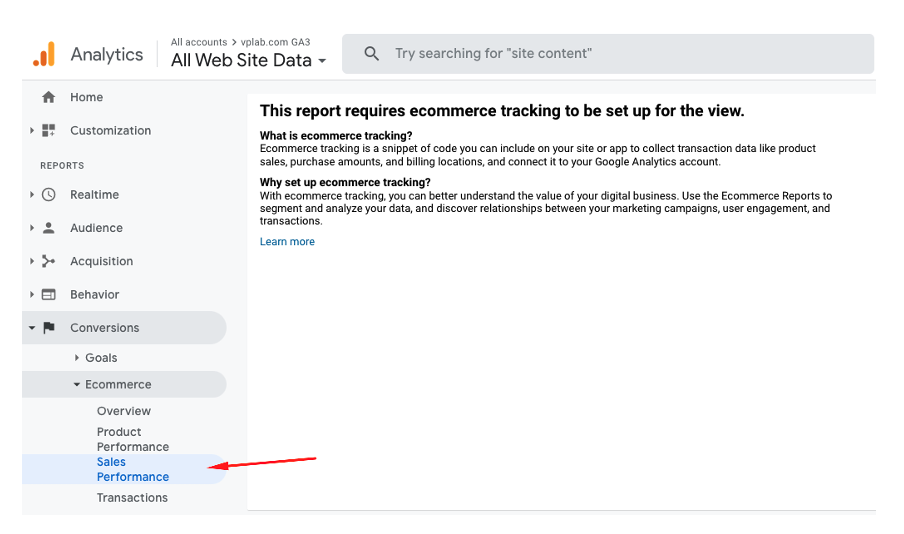Screenshot Description of a Website Analytics Page

This is a detailed screenshot of a website analytics dashboard. On the left-hand side, there is a vertical menu. At the top of the menu, there is an icon showing A signal strength, colored in red and orange, labeled as "Analytics" in black text. Below this, in grey text, it says "All Accounts" accompanied by an arrow indicating a dropdown menu, listing "vplab.com" followed by "GA 3" in capital letters. 

Moving further down the left menu, in bold black text, it says "All Website Data" with a dropdown arrow. Below this, there is a dark grey section with a black magnifying glass icon; the text "Try searching for 'site content'" is written in dark grey next to it.

On the left-hand side again, there is a mid-grey section featuring a dark grey house symbol labeled "Home." Below that, there are three squares and a plus sign, representing "Customization" with an arrow next to it. Under this, a grey section is labeled "Reports."

Within the reports section, there are several subsections:
- An arrow next to a clock labeled "Real-Time"
- An arrow next to a person icon (a circle and half-circle) labeled "Audience"
- A triangle next to a share symbol labeled "Acquisition"
- A triangle next to a square labeled "Behavior"
- A dropdown next to a flag labeled "Conversions"
- An arrow next to "Goals"
- A dropdown next to an e-commerce icon

There is also a subsection with selected options in blue text labeled "Sales" and "Performance," highlighted by a red arrow pointing to it.

In the main part of the screenshot:
- "Transactions" is written in black text.
- Below this, there is a bold black text stating, "This report requires e-commerce tracking to be set up for the view."
- Following that, in bold black text, it says, "What is e-commerce tracking?"
- Regular black text explains, "E-commerce tracking is a snippet of the code you can include on your site or app to collect transaction data like product sales, purchase accounts, and billing locations, and connect it to your Google Analytics account."
- Another bold black heading asks, "Why set up e-commerce tracking?"
- Below it, in black text, "With e-commerce tracking, you can better understand the value of your digital business. Use e-commerce reports to segment and analyze your data, and discover relationships between your marketing campaigns, usage engagement, and transactions."
- At the bottom, there is a "Learn more" link in blue text.